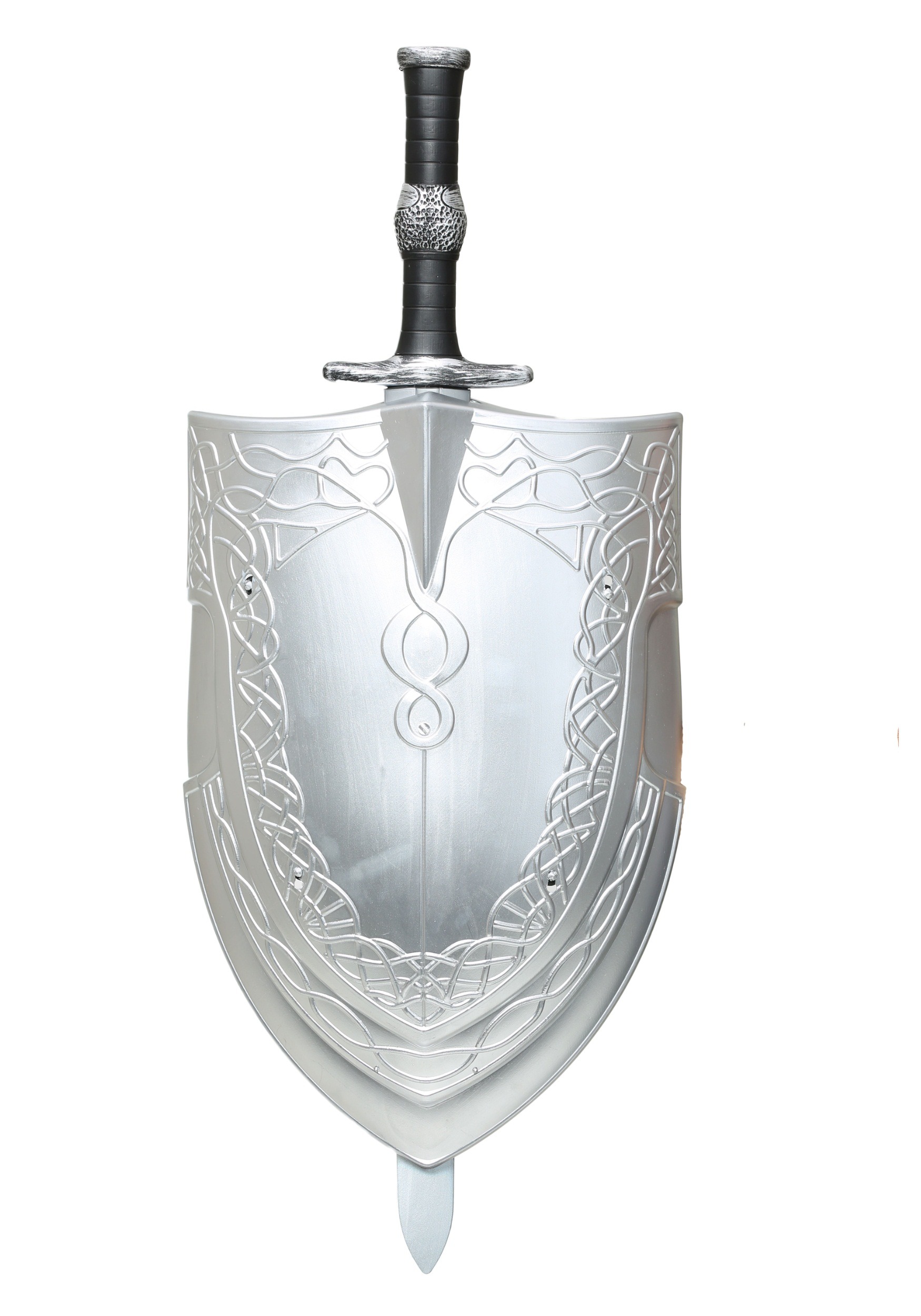The image showcases an ornate silver-colored shield with a sword positioned behind it, creating a striking combination. The shield, predominantly silver with intricate lines woven around its exterior, leaves a central plain spot that reflects white light. The top of the shield features the handle of the sword, which has a distinctive design: a black grip segmented by a silver ring adorned with black dots. The grip culminates in a silver circle at the very top. Below this, a silver guard extends to the sides, from which the blade descends. The blade itself is a light gray, tapering to a sharp point about a quarter of the way down the shield and reappearing at the bottom as the tip of the knife. The entire setup is set against a plain white background, highlighting the detailed craftsmanship of both the shield and sword, which together appear as part of a Halloween costume.